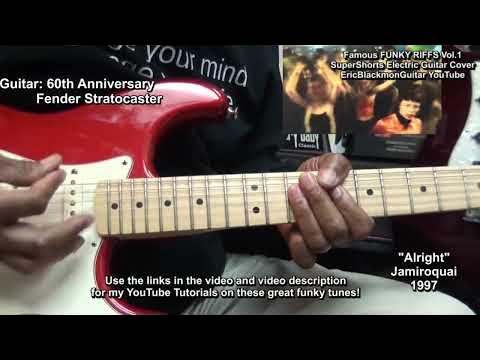The image is a detailed, color photograph in landscape orientation featuring a close-up of a man playing a red Fender Stratocaster electric guitar. The guitar has a cream-colored pick guard and a light wood neck. The man is holding a pick in his right hand, strumming the strings, while his left hand grasps the neck of the guitar, forming a chord. He is wearing a black t-shirt with the white partial text "Your Mind" visible.

In the upper left corner of the image, white text reads "Guitar: 60th Anniversary Fender Stratocaster." The upper right corner features a smaller inset photograph, slightly out of focus, depicting a crowd with the overlay text "Famous Funky Riffs, Volume 1, Super Shorts, Electric Guitar Cover, Eric Blackmon Guitar, YouTube." At the bottom of the main image, white text instructs viewers to "use the links in the video and video description for my YouTube tutorials on these great funky tunes."

In the lower right corner, additional white text reads '"Alright," Jamiroquai, 1997.' The image emphasizes a realistic, photographic style with textual elements providing context and promoting YouTube guitar tutorials.